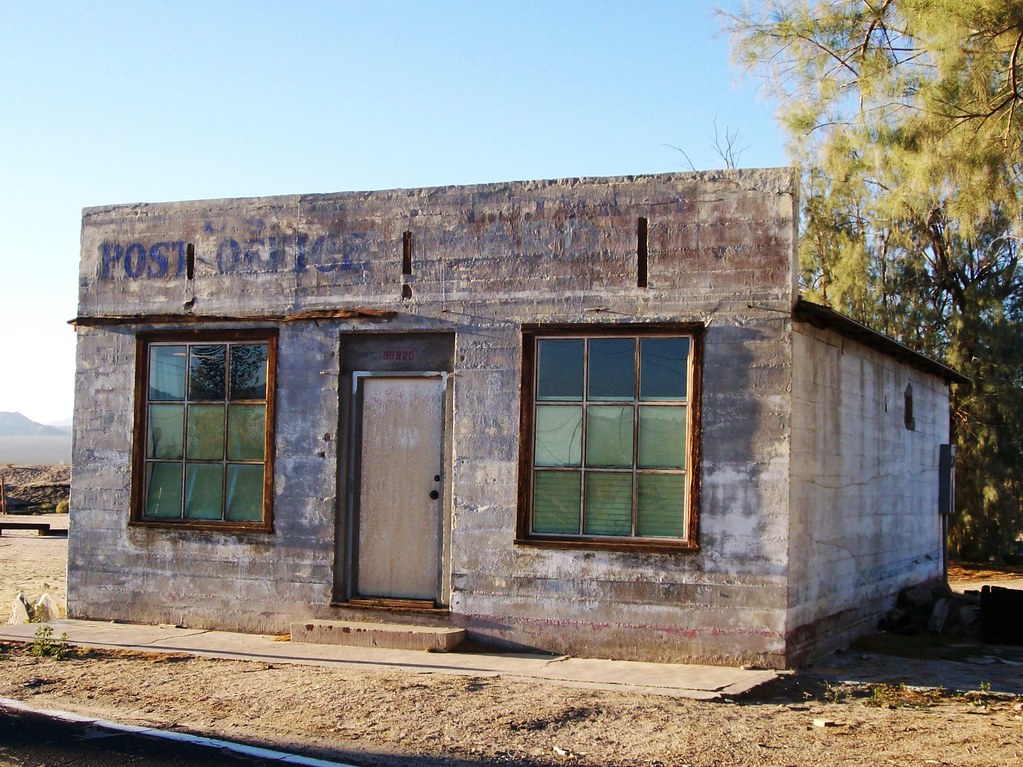The photograph captures an old, dilapidated building that was once a post office, nestled in what seems to be a deserted town. The small cement block structure features a disheveled appearance, with its paint fading and its upkeep clearly neglected. "Post Office" is faintly visible in blue font on the upper left side of the building. The doors and windows, although still intact, are partially covered with paper, obscuring the view inside. The shack is surrounded by a barren landscape of dirt paths with a couple of trees and rocks scattered nearby. A railroad track lies directly in front of the building, and in the background, a couple of additional roofs can be spotted under a light blue sky. The building, positioned out in the middle of nowhere, stands alone in an area devoid of life, as its surrounding dirt paths meander aimlessly, ending abruptly at nothing.